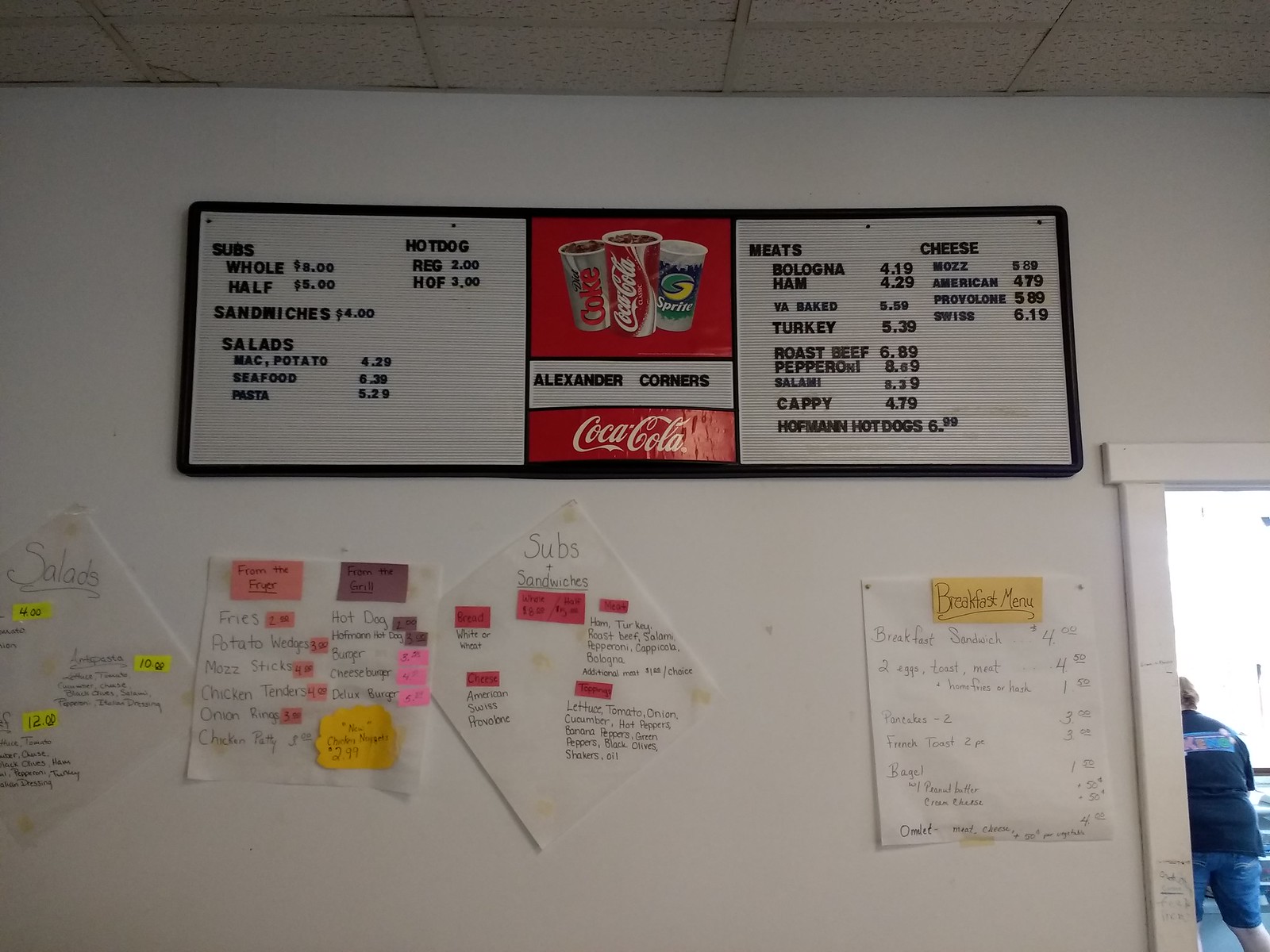This photograph captures the vibrant and eclectic feel of a cozy deli or restaurant. The upper portion of the image showcases a white wall adorned with a classic beige office tile ceiling. Prominently displayed at the top of the wall is a marquee-style sign, framed in black. The sign features a red section at the bottom which proudly displays the Coca-Cola logo in white. Above this section, three cups brimming with ice and liquid advertise Diet Coke, Coca-Cola, and Sprite. Centrally located on the marquee sign, "Alexander Corners" indicates the establishment's name.

Flanking the name on both sides are neatly categorized menu items – on the left, "Subs", "Sandwiches", "Salads" alongside "Hot Dogs", and on the right, "Meats", "Cheese", and additional "Hot Dogs", each section listing prices for the items.

Beneath this marquee sign are four separate pieces of white paper taped to the wall using clear tape. The first piece on the right is a rectangular white paper with a yellow attachment labeled "Breakfast Menu" featuring handwritten items and prices in pencil. This menu includes breakfast staples like breakfast sandwiches, French toast, and bagels.

In the center, a diamond-shaped white sheet is labeled "Subs and Sandwiches." This paper creatively utilizes red post-it notes to print sandwich names, with handwritten descriptions beneath each name in pencil.

To its sides are additional pieces of paper listing side items such as fries, potato wedges, mozzarella sticks, chicken tenders, and onion rings. The final paper, also in a diamond shape, is dedicated to different salad offerings, complete with descriptions and prices.

This detailed and homely display offers a glimpse into the welcoming and unpretentious charm of Alexander Corners.